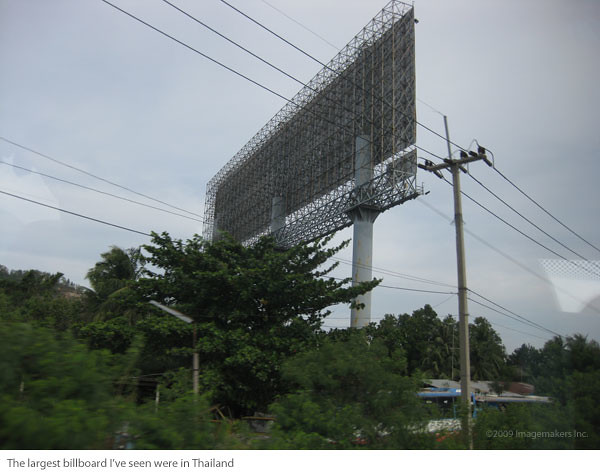In this photograph, the largest billboard I've ever seen, reportedly located in Thailand, dominates the composition. The billboard's massive frame is centrally positioned but faces away from the viewer, angled toward the upper left corner of the image. It is held up by gray supporting poles that match the overcast sky, which is suffused with subtle, indistinct clouds. 

In the foreground, a swath of lush green trees creates a stark contrast against the industrial elements. Intersecting the greenery, several power lines stretch diagonally from the top left to the bottom right of the frame, connected to a singular power pole situated to the right of the billboard. Amidst the foliage in the distance, small, weathered buildings in shades of gray, brown, and blue peek through, adding a touch of human presence to the scene. At the bottom left corner of the photograph, there is a text caption reading, "the largest billboard I've ever seen were in Thailand," left without any punctuation.